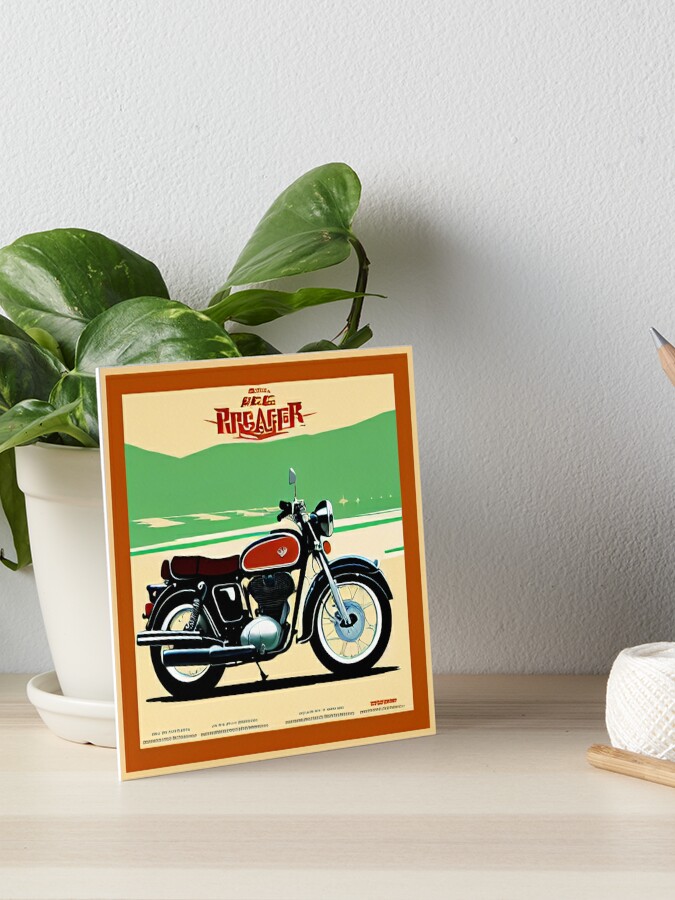The image depicts a small, framed sketch of a motorcycle viewed from the side, with the front tire facing right and the back tire left. The motorcycle features a prominent British orange gas tank, black tires with black rims, a red/orange reflector at the front, a muffler at the bottom left, and a visible kickstand. The scene within the sketch shows the motorcycle on a light beige sandy area set against light green hills under a yellowish sky. Above the motorcycle, sophisticated and somewhat illegible red lettering begins with a "P," "S," or "R." The sketch is outlined first by an orange frame and then a yellow one.

The framed image is propped up against a white terracotta pot containing a large fig leaf plant. Surrounding this scene is a light wood surface, and behind it, a soft gray or black-and-white plaster wall. Off to the right, there is a ball of string or yarn, a wood stick, possibly used for embroidery or fine crochet, and a pen or pencil in an upright container.